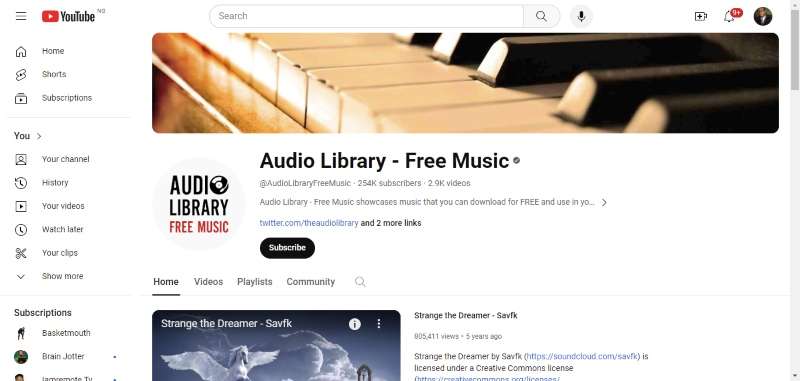The image displays the YouTube home webpage, predominantly featuring a clean, white interface. On the left-hand side, a vertical navigation menu is visible, containing several sections such as 'Home,' 'Shorts,' and 'Subscriptions.' Below these, the 'You' section includes options for 'Your channel,' 'History,' 'Your videos,' 'Watch later,' 'Your clips,' and a 'Show more' link presumably offering additional features. This menu also lists the channels the user is subscribed to.

Centered prominently on the page is a rectangular image of a piano positioned just beneath the white search bar. This image is associated with the 'Audio Library Free Music' channel, indicating the presence of free music content. The highlighted 'Home' section currently displays a thumbnail for "Strange the Dreamer," which is likely a song provided by the channel. 

The top-right corner showcases the user account's logo, where account-related features and settings are accessible. Overall, the image captures the key navigational and visual elements of the YouTube home webpage.